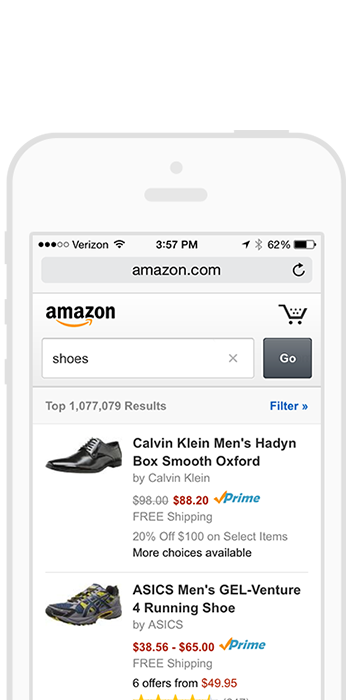This is a detailed screenshot displaying a phone mock-up featuring an Amazon.com page. The phone's screen showcases a search for "shoes" on Amazon. 

At the top of the screen, there is a gray navigation bar displaying the URL, with a refresh button on the right. Below that, the Amazon logo is prominently shown on the left, accompanied by a shopping cart icon on the right. 

Underneath, a white search bar containing the word "shoes" occupies the screen, flanked by an "X" to clear the search and a square gray "Go" button. Following this, a light gray bar indicates that there are "Top 1,077,079 results" with a blue "Filter" link on the right.

The search results section displays two listings for shoes. The first entry is "Calvin Klein Men's Hayden Vox Smooth Oxford," featuring a thumbnail image of the shoe on the left. To the right of the thumbnail, the listing details include the title, name of the maker, price, and available shipping options.